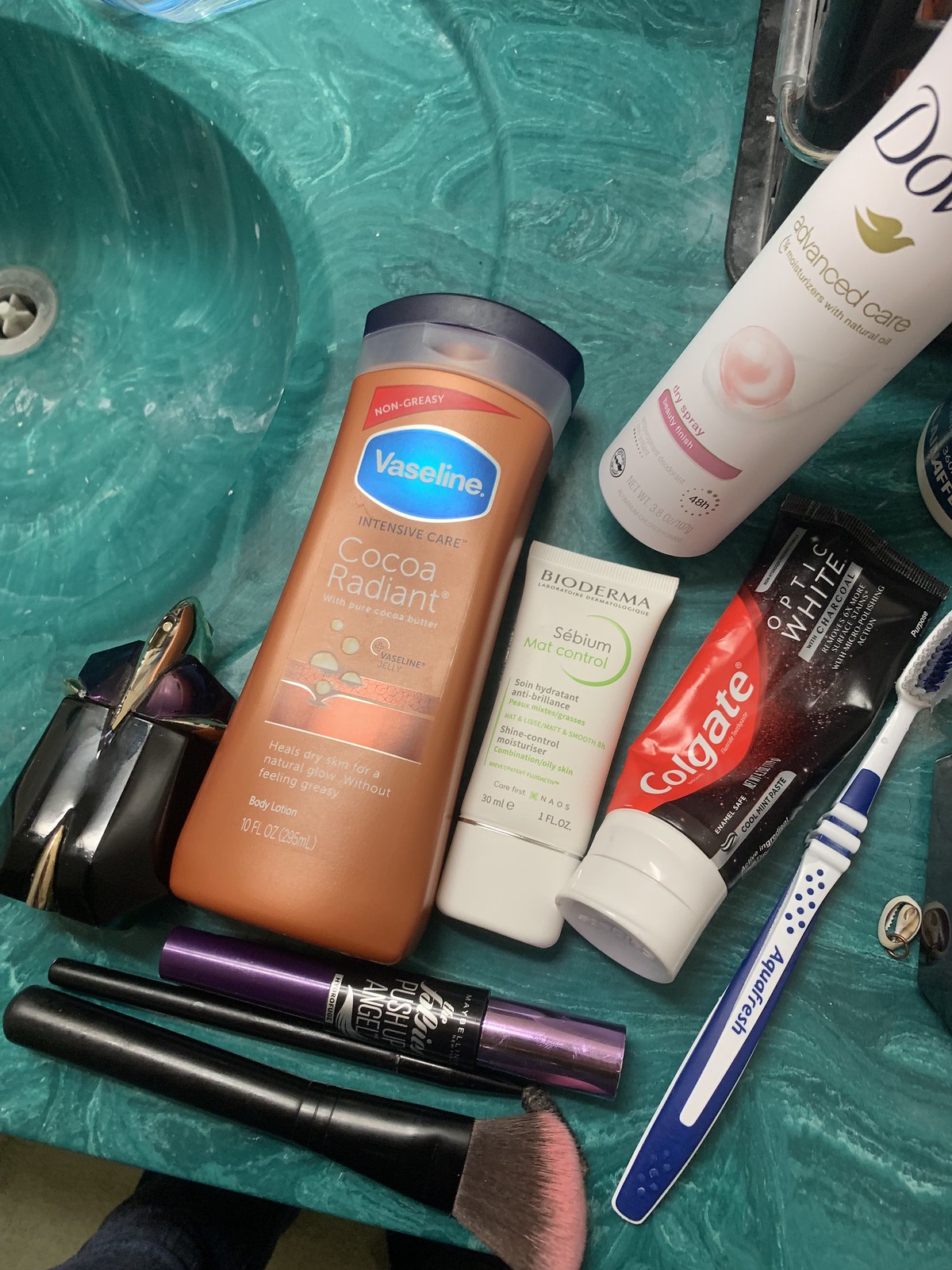On a marbled teal-blue countertop, which matches the texture and color of the adjacent sink, lies a collection of typical bathroom implements. The silver drain at the center of the basin, complete with a white plug, is visible to the left of the scene. In the top right corner, part of a black plastic container is just visible. 

In the bottom left corner of the frame, beyond the counter, a person’s blue-jean-clad leg can be seen. 

On the counter, starting from the bottom, there is a brush with a black handle and brown bristles tipped in pink. Above this, there is a black pen-like object, alongside a purple lipstick or similar item, labeled in silver text as "Push-Up Angel" from Maybelline. 

Above these items sits an orange bottle with a blue logo bearing the brand Vaseline. The text on the bottle reads: "Non-greasy intensive care, cocoa radiant with pure cocoa butter, Vaseline jelly. Heals dry skin for natural glow without feeling greasy. Body lotion, 10 fluid ounces, 295 milliliters."

To the right of this bottle is a white squeeze bottle with black text that reads: "Bioderma Sebium Matte Control, shine control moisturizer, combination/oily skin," followed by a repetition of this information in French. 

Nearby is a black tube of toothpaste with a red Colgate logo. Above these, a white bottle reads "Dove Advanced Care" and mentions "moisturizers with natural oil." To the right of all these products is a white and blue toothbrush.